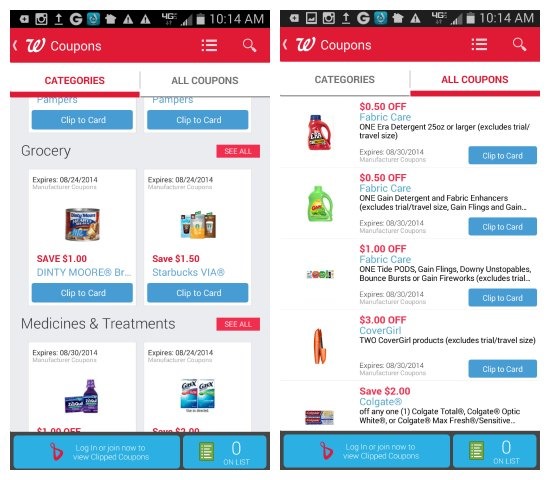Here is a descriptive and cleaned-up caption for the image:

---

The image is a screenshot from a mobile device, showcasing two different couponing screens. 

**Left Screen: Categories Tab**
- **Top Bar Icons:** Battery with a plus, camera, upload arrow, 'G', blue square, home, two caution triangles with exclamation marks, '4G', service at half strength, nearly full battery, and the time 10:14 AM.
- **Navigation Bar:** Red bezel featuring a left-pointing bold white arrow, a bold white ‘QW’ swirl, the text "Coupons" in white, a settings hamburger menu, and a magnifying glass icon.
- **Tab Selection:** "Categories" tab highlighted in red with an underline; "All Coupons" tab in grey.
- **Coupon Listings:** 
  - "Pampers": Save on Pampers products with a "Clip to Card" dark blue button.
  - "Grocery": Highlighted under a dark grey section with a prominent "See All" red button. Featured item includes a Del Monte can with "Save $1" in red and "Denti Mori" in cyan blue, and "Clip to Card."
  - Other items include Starbucks products with $1.50 off, cough syrup with $1 off, and juice boxes with $3 off.

**Right Screen: All Coupons Tab**
- **Tab Selection:** "All Coupons" tab selected, featuring a detailed list of various items.
- **Coupon Listings:** 
  - Laundry detergent (orange with blue cap): "$0.50 off" in red, "Fabric Care" in cyan, detailed item description in black, with expiration date "08/30/2014" in grey.
  - Gain detergent (lime green): "$0.50 off" in red, "Fabric Care" in cyan, detailed text partially cut off, with expiration date "08/30/2014."
  - Tide Pods: "$1 off" in red, "Fabric Care" in cyan, detailed text partially cut off.
  - Other items include Covergirl cosmetics with $3 off, and Colgate toothpaste with $2 off, each detailed with restrictions and formatted in red and cyan blue text.

Both screens emphasize the "Clip to Card" feature for coupons for easy online shopping benefits.

---

This cleaned-up version provides a detailed breakdown of the key elements and text within the screenshot, giving a clear understanding of the layout and content.